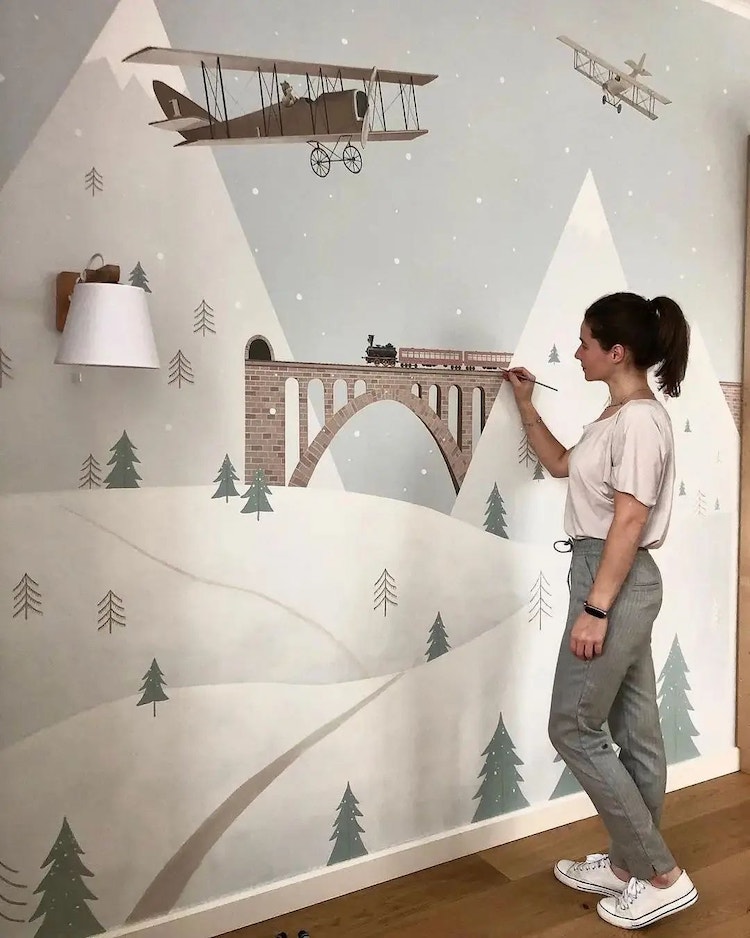In this carefully staged, full-color vertical photograph, we find ourselves indoors with a clear view of a wooden floor. Dominating the right side of the image is a young woman with shortish, dark brown hair pulled back into a ponytail. She wears a white, short-sleeved shirt tucked into gray sweatpants and white tennis shoes, notably without visible socks. With a paintbrush in hand, she focuses intently on a large mural on the wall.

The mural she is creating exudes a whimsical, wintry scene. At the forefront, snowy hills and pine trees stretch across the canvas, framing two prominent, pointy triangular mountains. Nestled between these mountains is a distinctive brick bridge with a large archway, leading into a tunnel at the base of one of the peaks. Above the idyllic landscape, a pair of vintage biplanes soar through the sky.

Her artistic style leans towards a charming, child-friendly motif, distinctly non-photorealistic, evoking the playful essence of a scene suited for a kid's room. Despite mentions of disparate elements like a white man attached to a wall or Chinese mountains, these elements do not visually manifest in the image provided, allowing the mural and the woman’s focused artistry to remain the central points of attention.